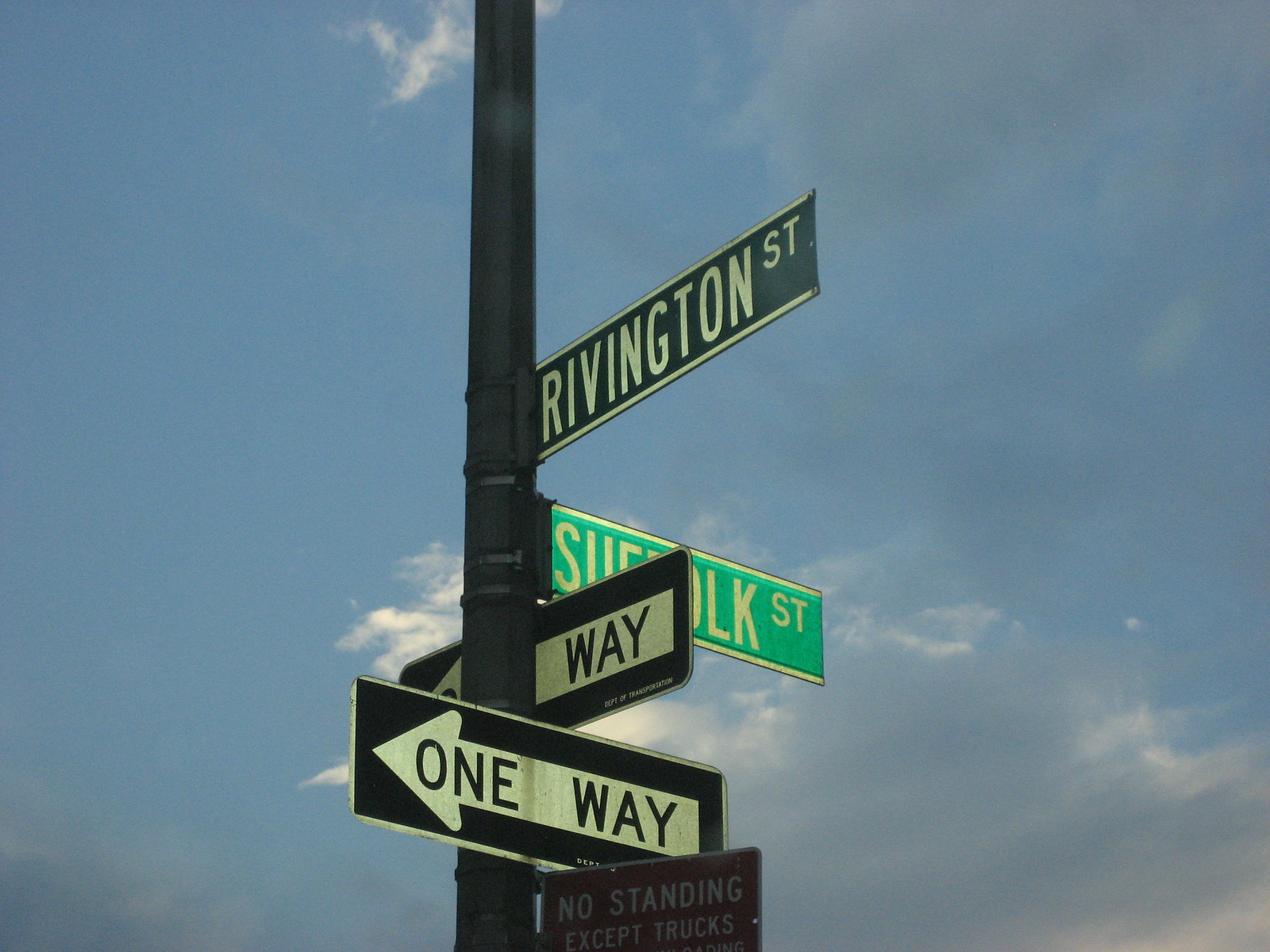The image captures an urban street scene centered on a metal light pole against a backdrop of a clear blue sky scattered with a few small white clouds. The light pole, whose full height is not visible as both the top and the bottom extend out of the frame, prominently displays several signs. At the top, there's a green street sign labeled "Rivington Street." Below this, another green street sign indicates "Suffolk Street," facing the opposite direction. Underneath these street signs, two white "One Way" signs are attached; the top one points to the left, and the one beneath it also points left but at a sharper angle. Further down, there is a small red sign that reads "No Standing Except Trucks," though the remaining text on this sign is obscured and unreadable. The composition highlights the functional aspects of city infrastructure amidst an open sky, implying a bustling urban environment.